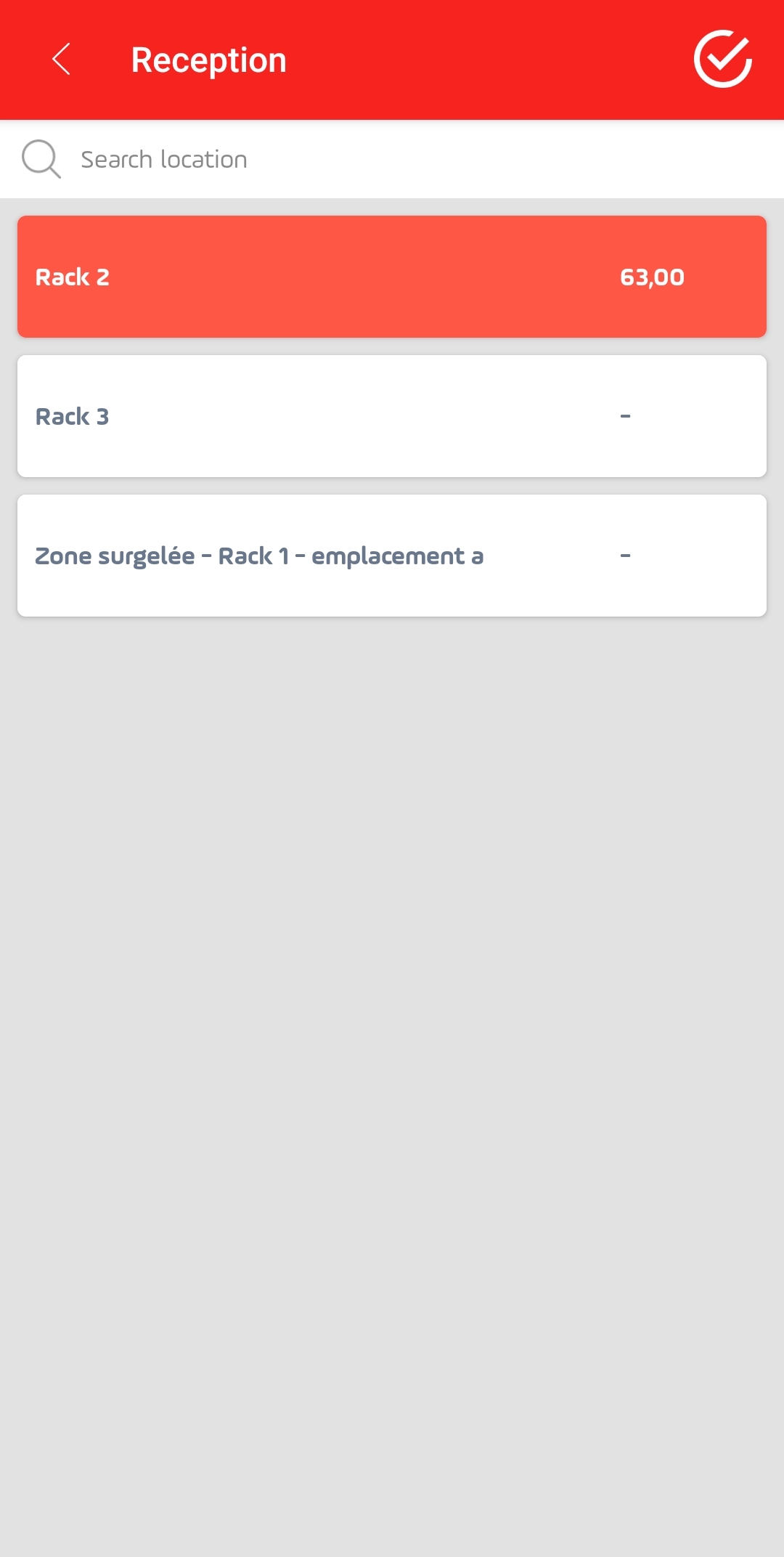This is a detailed screenshot from a mobile interface. The image appears to be cropped and features a vivid red header at the top. On the left side of the header, there is a white arrow pointing to the left. Just to the right of this arrow, the word "Reception" is displayed in small white letters. Located in the top right corner of the red header, there is a white checkmark enclosed in a white circle.

Following the header, still within the upper section, there's a prominent white search bar. On its left side, there is a small magnifying glass icon. Adjacent to this icon, in small gray letters, it reads “Search location.”

Beneath the search bar, the main section contains three rectangular information boxes. The first box stands out with its red color. On the left side, it indicates “Rack Two” in small white letters, and on the right side, it lists a price of "$63.00."

The second rectangular box is white and simply states “Rack Three” on the left, while the right side contains only a small dash, indicating no value or item.

The third and final white box is more descriptive. It reads “Zone Serge Lay - Rack One - Placement A” on the left side, though the right side also features just a small dash, similar to the second box.

The background of the screenshot is gray and devoid of any other details or information.